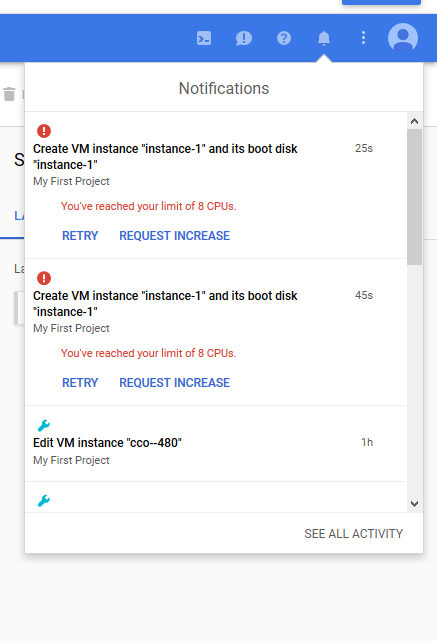A detailed screenshot captures the notifications panel of a desktop software interface. The header at the top of the screen is light blue, and several icons are aligned on the top right, including information, questions, and alert icons. The alert icon has been selected, unveiling a notifications box overlaying the screen's background.

The notifications box is titled "Notifications" in gray at the top. The first alert showcases a red exclamation mark icon on the top left, followed by a bold message: "Create VM instance (instance 1)," and in smaller font, "its boot disk (instance 1)." Below this, in gray text, is "My First Project." A warning in small red font states: "You've reached your limit of eight CPUs." The options "Retry" or "Request Increase" are presented in capitalized blue letters below this warning.

The second alert mirrors the first, displaying the same red exclamation mark icon and message: "Create VM instance (instance 1) and its boot disk (instance 1)."

The third alert features a blue wrench icon. Below it, in text, it reads: "Edit VM instance CCO--480." At the alert's bottom right corner, the option "See all activity" is shown in bold gray font.

This detailed panel provides essential alerts and actions for managing VM instances within the project.